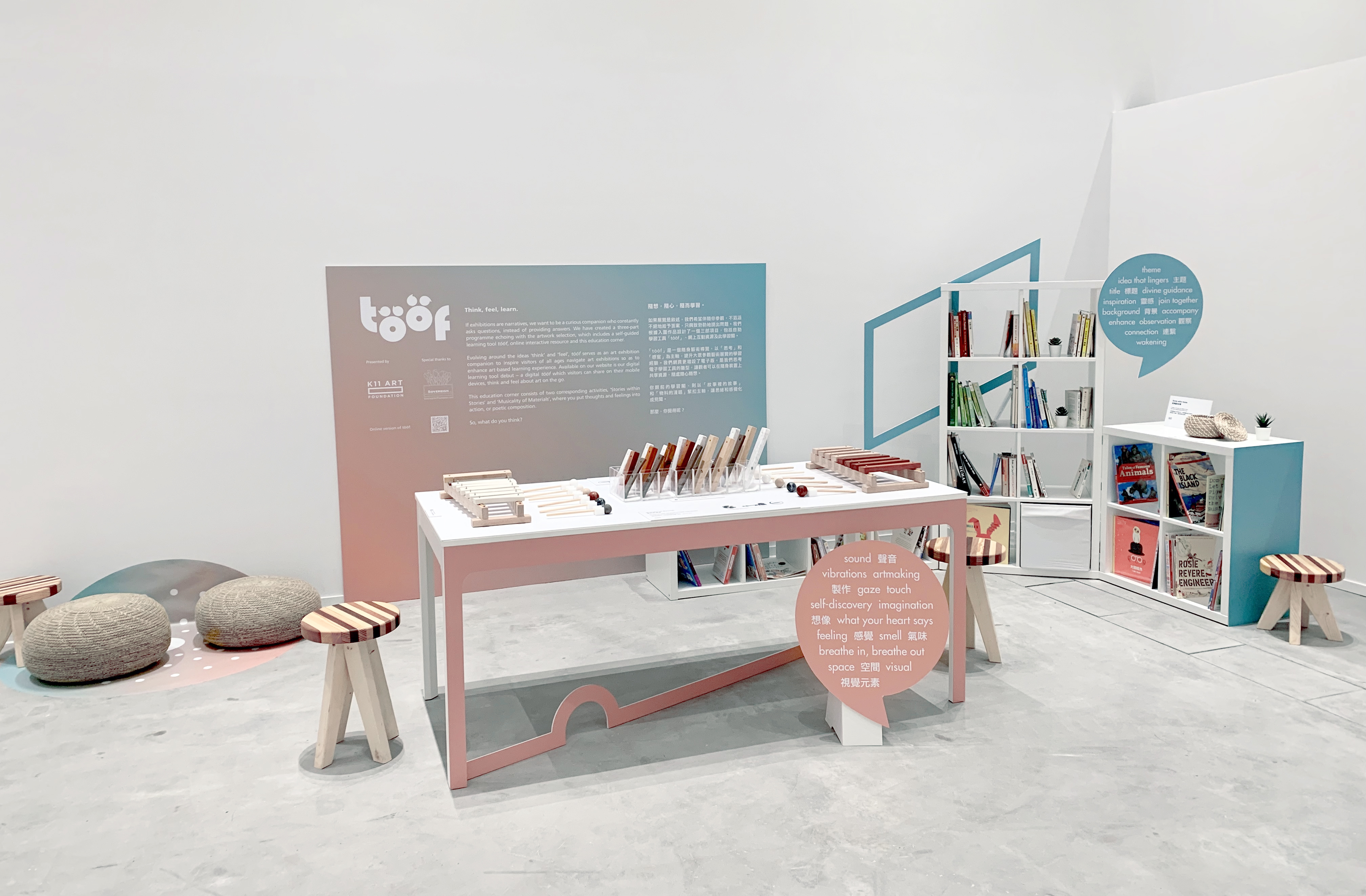The photograph showcases a modern, white-walled art room filled with various creative and learning materials. Dominating the back of the room is a large banner with a logo that reads "T.O.O.F." alongside other smaller, indecipherable text. The room's centerpiece is a long table with a white top and a pink front, which is scattered with art supplies. Adjacent to the table, a sturdy, three-legged wooden stool with dark, striped wood on its top surface adds to the room's eclectic furnishings. On the left side of the room sit some beanbag seat cushions, while the back right corner features a set of bookshelves filled with books and topped with another wooden stool. Much of the furniture, including the bookshelf, has blue and pink framing, complementing the overall white and clean aesthetic of the room.